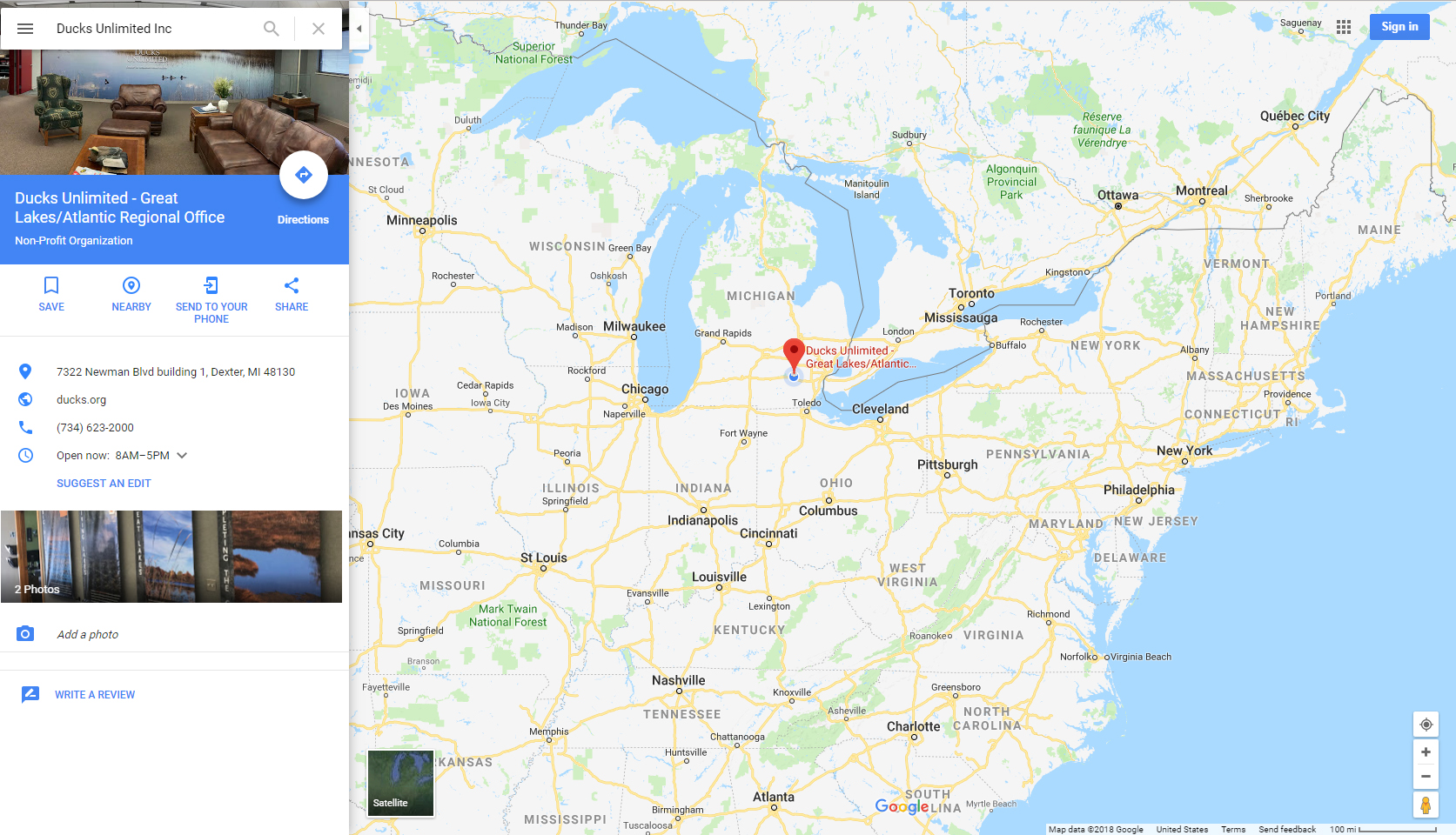This image is a color screenshot from a computer screen, showcasing a Google Maps view in landscape format. The left side features the details of Ducks Unlimited Great Lakes Atlantic Regional Office, located at 7322 Newman Boulevard, Building 1, Dexter, Michigan, 48130. Visible elements include its name, website (ducks.org), phone number (734-6232), and operating hours (8 a.m. to 5 p.m.). Below this information, there are action buttons for "Save," "Nearby," "Send to your phone," and "Share," followed by a collection of clickable photos. The right side displays a large map of the eastern United States, extending from the central U.S. to Maine and down to around Atlanta, highlighting the office's precise location with a red marker. Major states and cities are labeled to provide a clear sense of geographical context.